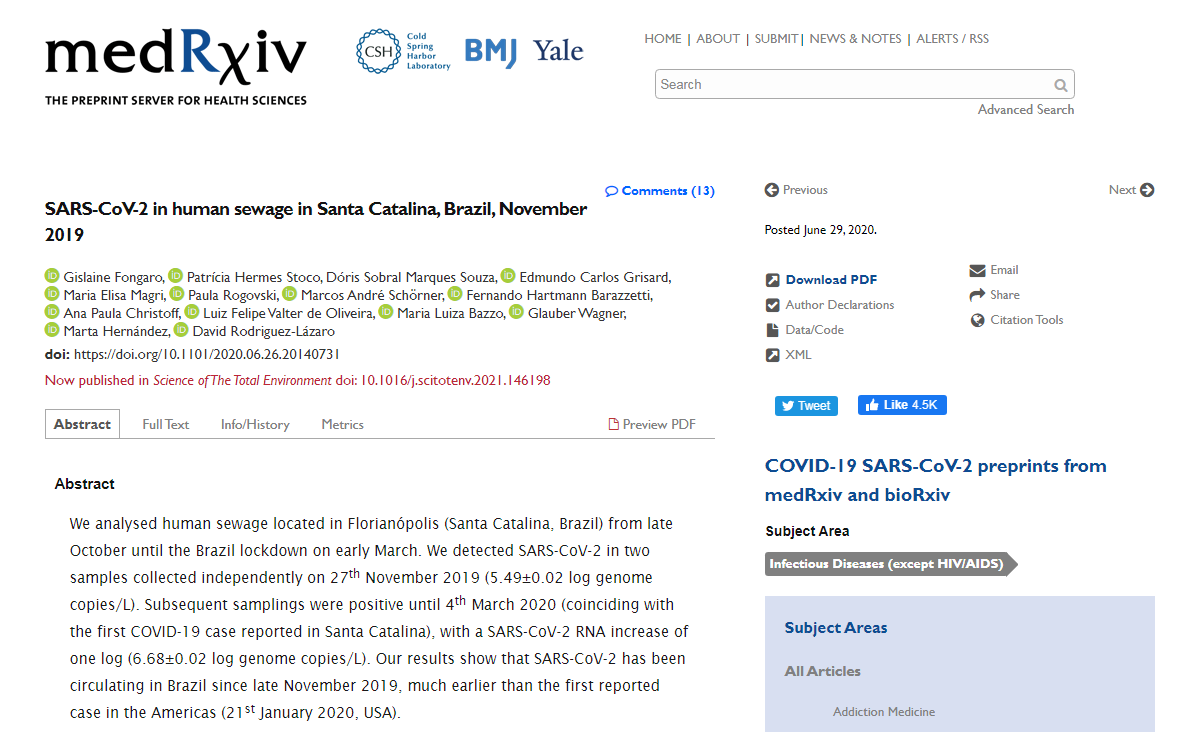This image showcases a detailed screenshot of a webpage from MedRxiv, affiliated with CSH Cold Spring Harbor Laboratory. Iconography includes logos like BMJ and YEL. The navigation bar contains various options such as Home, About, Submit, News and Notes, Alerts/RSS, and features a search box with a gray magnifying glass icon.

Prominently displayed is the title "SARS-CoV-2 in Human Sewage in Santa Colita, Brazil, November 2019," followed by an extensive list of author names and their respective IDs. It is noted that the research has been published in "Science of the Total Environment."

The main body of the page contains the abstract, beginning with the highlighted word "Abstract." The study describes an analysis of human sewage in Santa Colita, Brazil, from late October 2019 until the country’s lockdown in early March 2020. Researchers detected SARS-CoV-2 in samples collected independently on November 27, 2019, through March 4, 2020, aligning with the first reported COVID-19 case in Santa Colita. The findings indicate a significant increase in SARS-CoV-2 RNA, with a measured surge of 1 log 6.68 ± 0.02 log genome copies, suggesting that the virus was circulating in Brazil much earlier than the first reported cases in the Americas on January 21, 2020.

The page predominantly features a white background with black text. Various interactive buttons are available, including options to tweet the page or like it on Facebook, giving it the functional appearance of a typical modern webpage.